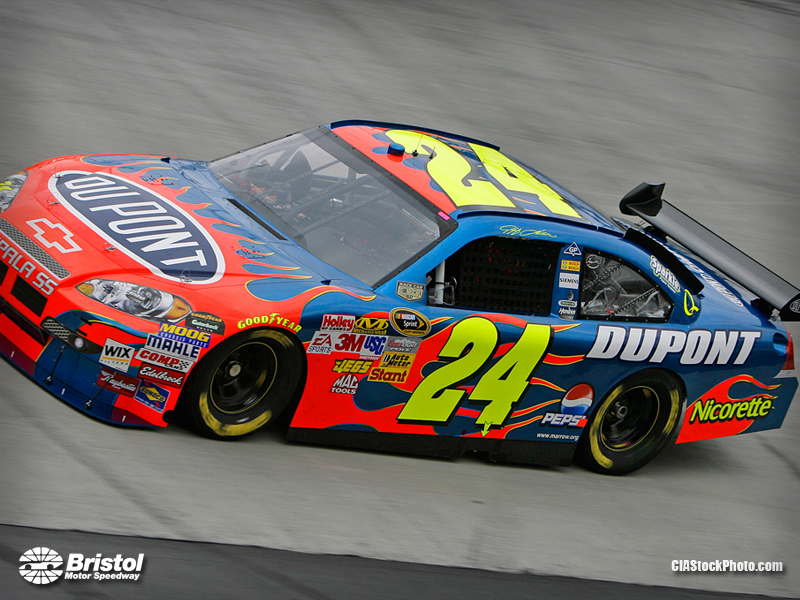The photograph captures a dynamic scene of a race car, predominantly blue with striking red and orange flames adorning the hood and sides, creating a sense of speed and intensity. The car proudly displays the number 24 in bright yellow on both the door and roof, making the racer easily identifiable. Above the back tire, 'DuPont' is prominently featured in white font, and the hood showcases a large blue oval with 'DuPont' in white text, emphasizing the primary sponsor. Additional sponsor logos, including Goodyear, Nicorette, Pepsi, Stant, Mac Tools, Jags, 3MUSG, Collery, EA Sports, Mahle, Comp, and Wix, are scattered across the car, particularly near the front tire and along the body. The vehicle's black tires, with white lettering in motion, and a visible roll cage with metal bars inside, highlight its readiness for high-speed racing. The car is captured while driving on a paved track, angled slightly to convey movement, with background text marking the venue as Bristol Motor Speedway. The bottom corners of the photograph bear the text 'CIAstockphoto.com' on the right and 'Bristol Motor Speedway' on the left, providing context and source information.